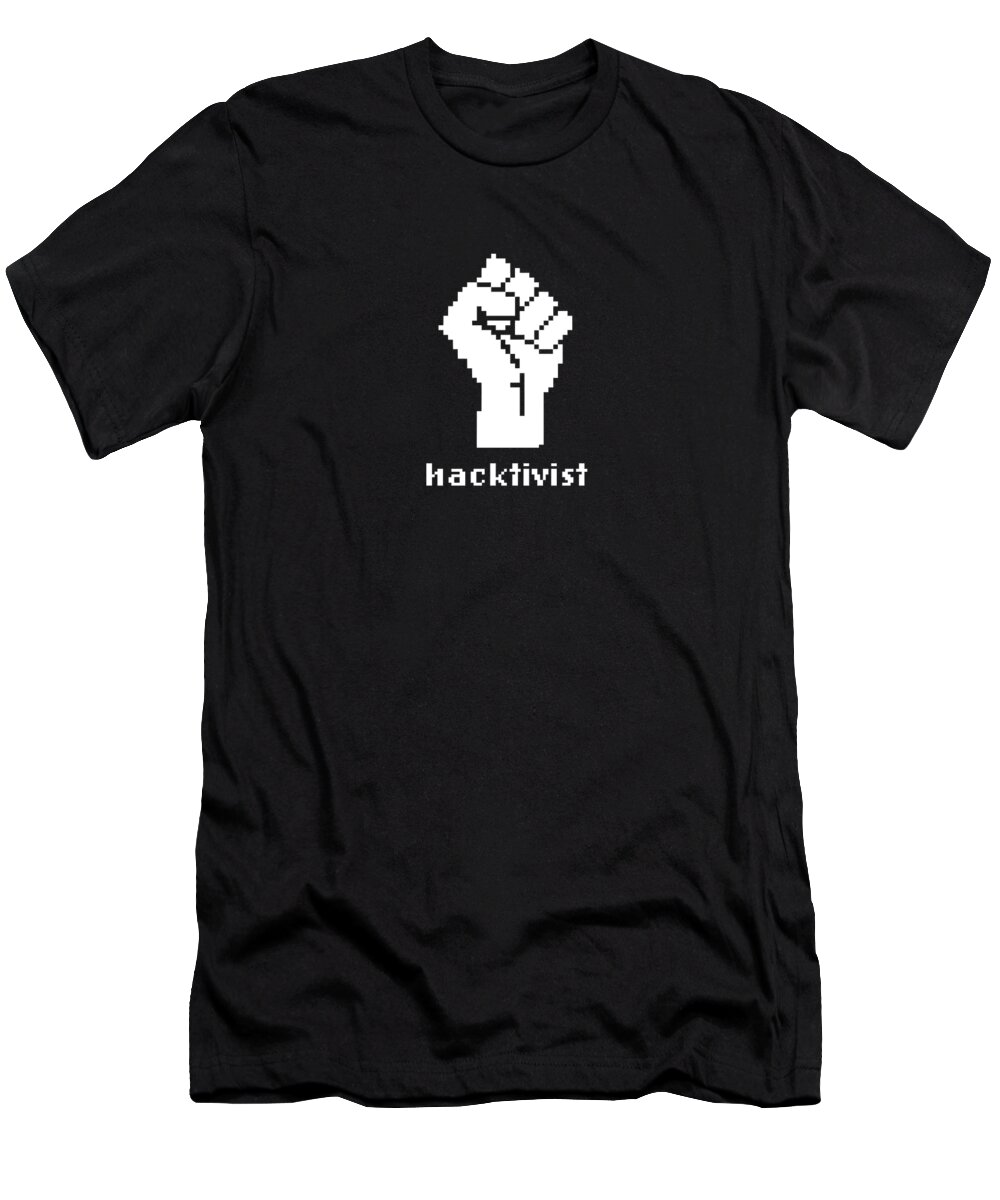In the image, a black, slightly wrinkled and ruffled short-sleeved crewneck t-shirt stands vertically against a white background. This simple t-shirt features a striking white graphic prominently centered on the chest. The graphic depicts a closed fist with the thumb positioned over the four fingers, palm facing forward, and detailed with black outlines. Below the fist, in bold white text, is the word "HACKTIVIST," spelled out as H-A-C-K-T-I-V-I-S-T. This is the sole design on the otherwise plain black t-shirt, creating a powerful and minimalist visual impact.